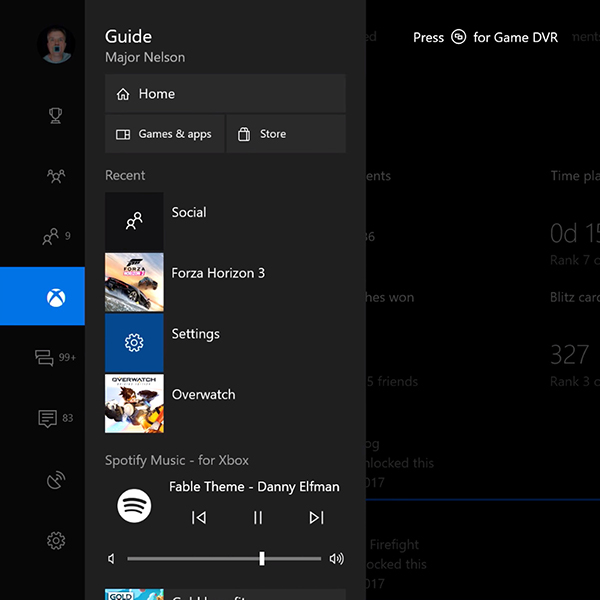The image depicts the main menu interface of an Xbox console. The central element is a large dialogue box with a black background labeled "Guide" at the top, followed by the name "Major Nelson." Below this label are three main navigation buttons: Home, Games & Apps, and Store. Beneath these buttons are four thumbnails representing different sections: Social, Forza Horizon 3 (a racing game), Settings, and Overwatch.

Further down, there is an area displaying currently playing music on Spotify, featuring the Spotify logo along with the track "Fable Theme" by Danny Elfman. This section also includes a progress bar and volume control.

To the left of the main dialogue box, various icons can be seen: a trophy button, a multiple-users button, and a dual-user button, with the Xbox button currently highlighted. Additionally, there’s a text message icon indicating 99+ unread messages, and another smaller dialogue box displaying the number 83.

Behind the dialogue box, there are hints of other gaming-related information partially obscured. In the top right corner, instructions mention pressing a specific button on the Xbox controller to activate the Game DVR feature. The overall background is predominantly black, creating a sleek and focused interface for navigating the Xbox system.